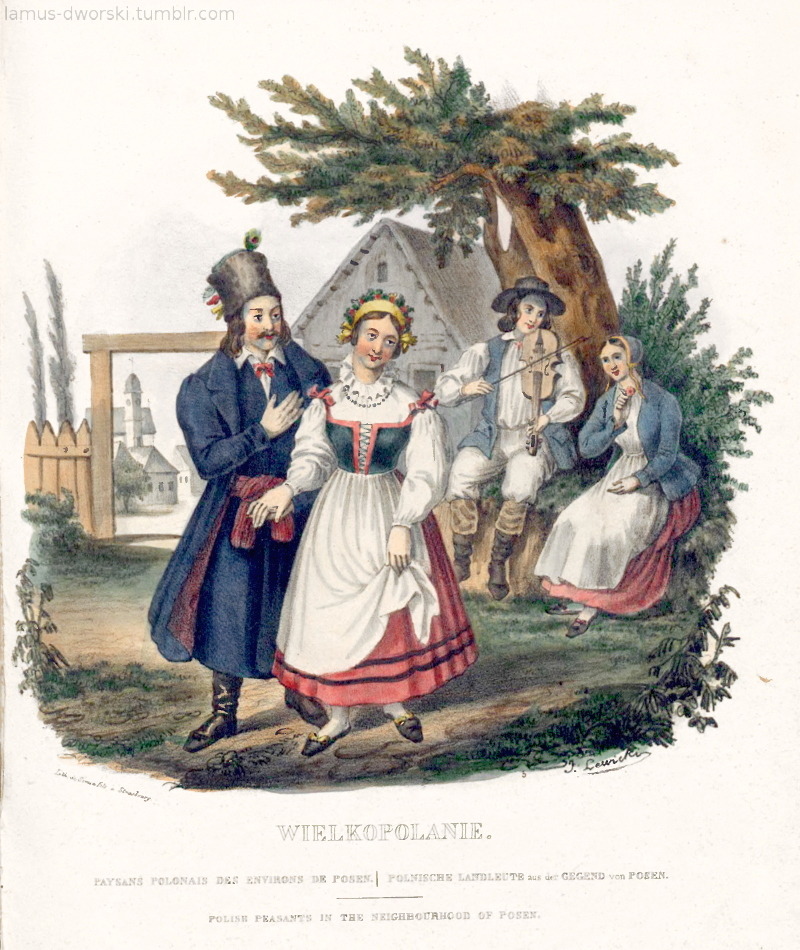A charming, rectangular painting, possibly taken from an old book or magazine, depicts an 18th-century courtship scene, measuring approximately 5-6 inches in height and 4-5 inches in width. The image, which includes text stating "L-A-M-U-S-D-W-O-R-S-K-I.tumblr.com" in light pink in the upper left-hand corner and "W-I-E-L-K-O-P-O-L-A-N-I-E" in black outline at the bottom center, portrays a colorful outdoor setting. 

A man, clad in a long blue coat that nearly reaches his ankles, stands poised in a traditional wide-brimmed hat adorned with a flower featuring yellow, red, and blue hues, as well as a peacock feather tip at the front. His attire is completed by a white shirt, a blue tie or blue vest, and a distinctly tied belt around his waist. Opposite him stands a Caucasian woman dressed in a vibrant red skirt with black stripes at the hem, a white apron, and a high-necked, ruffled white blouse. Her ensemble, tied together with red bows on the shoulders and adorned with a floral headband, exudes historical charm.

In the background, set against a rustic scene featuring a slanted roof house and a quaint brown gate leading into a village, a second couple enjoys a leisurely moment. The man plays a fiddle while the woman listens, seated under a tree. This lively, illustrative snapshot evokes the pastoral spirit of Polish peasants in the neighborhood of Posen, capturing a picturesque moment of joy and courtship.